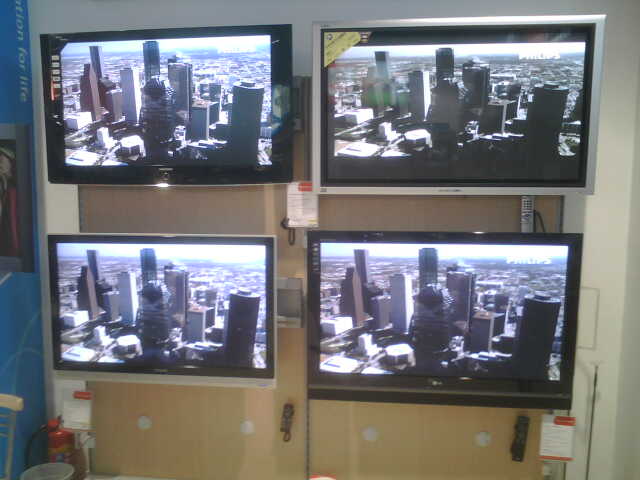The image features four brand-new Phillips TVs mounted in a square grid arrangement on a wooden door, seemingly set up to showcase their image quality in a store. Each TV displays the same daytime cityscape, featuring numerous skyscrapers from a high vantage point. The TVs vary in design: the upper left and lower right TVs have black bezels, while the upper right and lower left TVs have silver-colored bezels. Notably, the upper right TV has a yellow piece of paper in its top left corner, while red tags hang from three of the TVs (upper right, bottom left, and bottom right), indicating their prices. Adjacent to the setup, there is a bluish strip on the left side of the wall, and a fire extinguisher is visible on the floor.